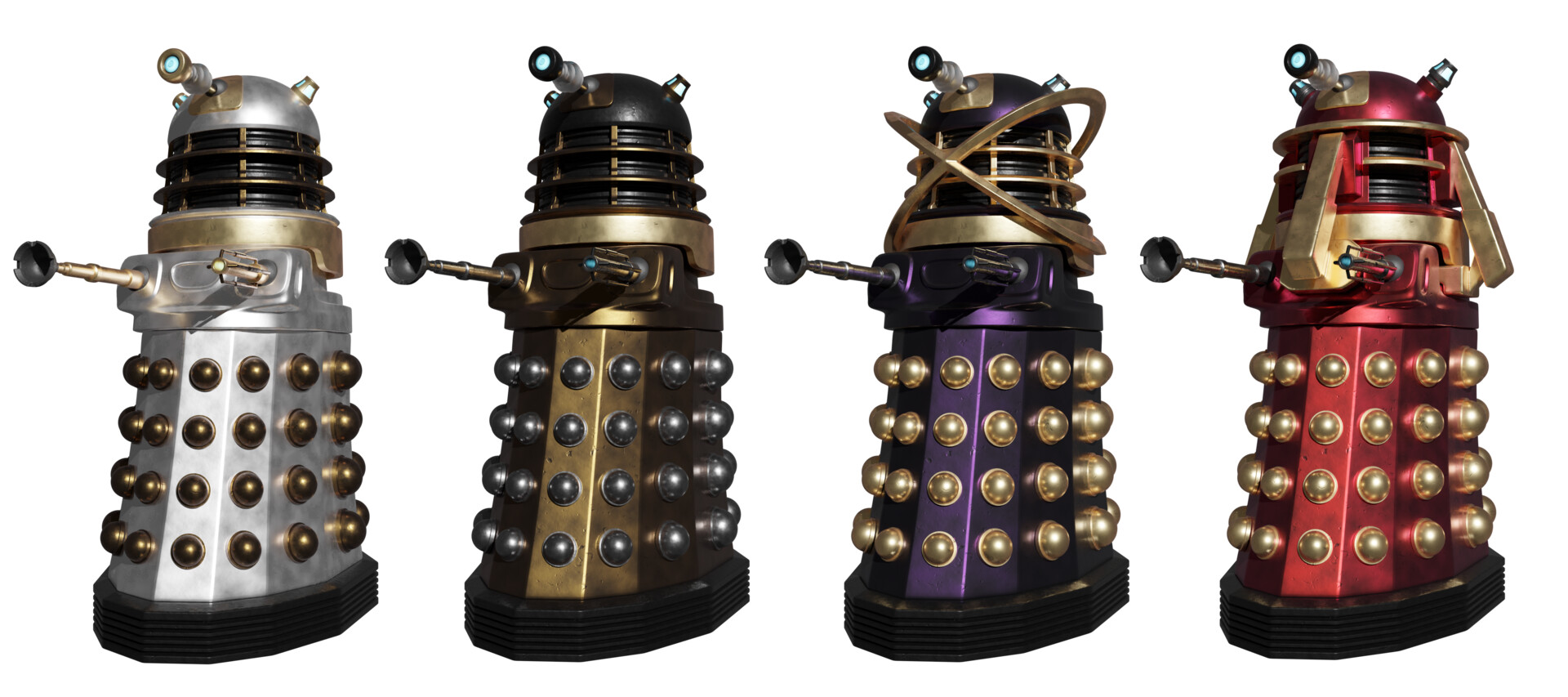This photo features four robots, each positioned side by side with even spacing against an all-white background. Each robot shares a similar shape, resembling a salt shaker with a round dome top and a faceted, polygonal cylindrical bottom. The robots are distinctly colored silver, dark brown, dark purple, and dark red. The bottom portions of the robots are adorned with rows of spherical protrusions aligned vertically in groups of four. Protruding from the body of each robot is an arm-like metal rod with a circular end. The top of each robot's dome is accented with an antenna-like feature. Additionally, these robots have either gold or silver decorative accents. The bases of the robots are black, giving an almost rubber bumper appearance. Notably, the purple robot features crisscrossing rings around its head. The overall design suggests these robots may serve a decorative purpose.